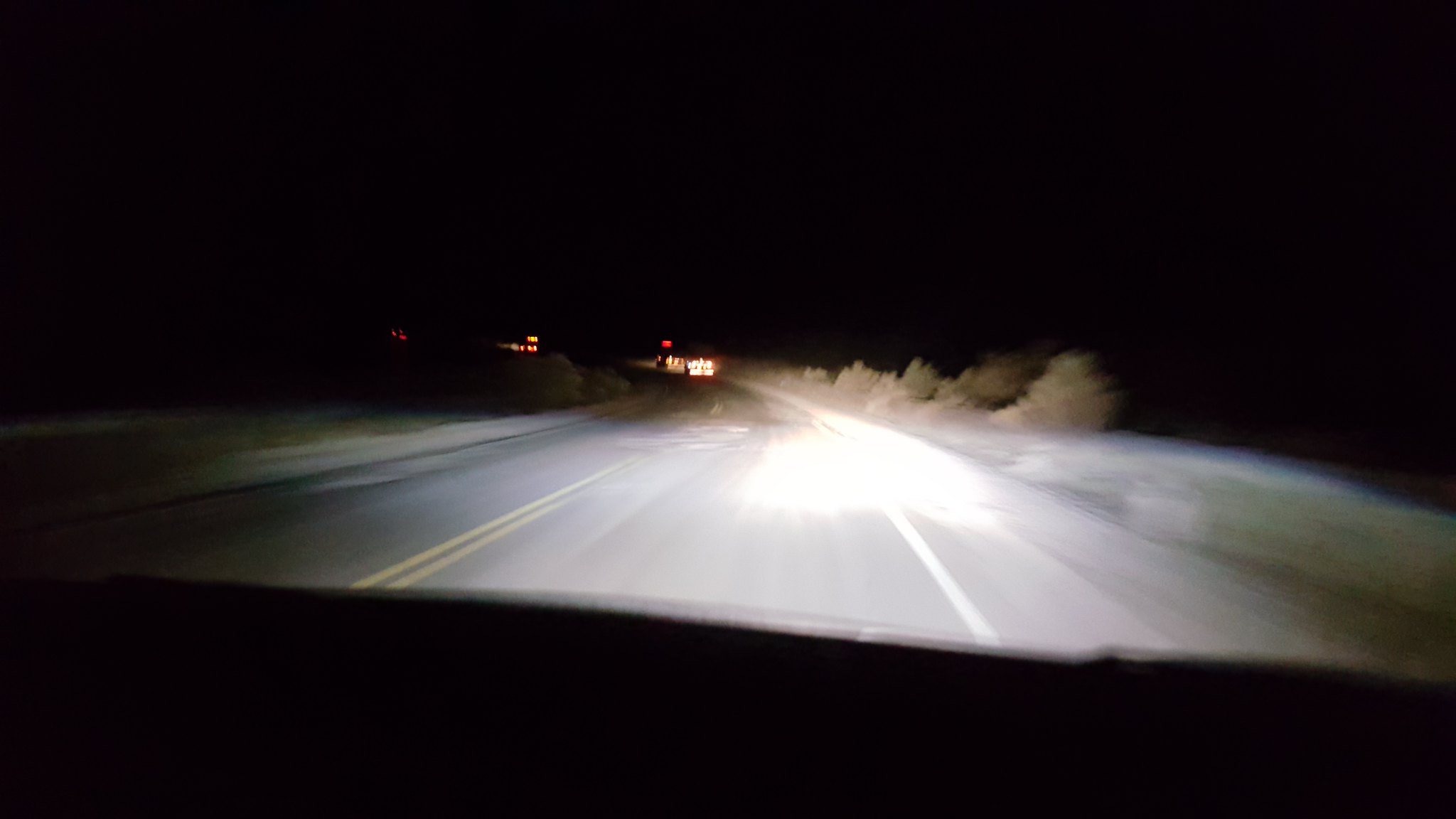A nighttime photograph captured through the windshield of a vehicle features a dark dashboard spanning the bottom edge. The view ahead reveals a pitch-black sky, with the vehicle's headlights casting light onto the gray road, marked by a double yellow line down the center. On the right shoulder of the road, clusters of light green, short plants and bushes are visible. In the distance, the rear lights of other vehicles punctuate the dark road, indicating the presence of fellow travelers at a considerable distance ahead. The composition conveys a sense of quiet, nocturnal journeying.